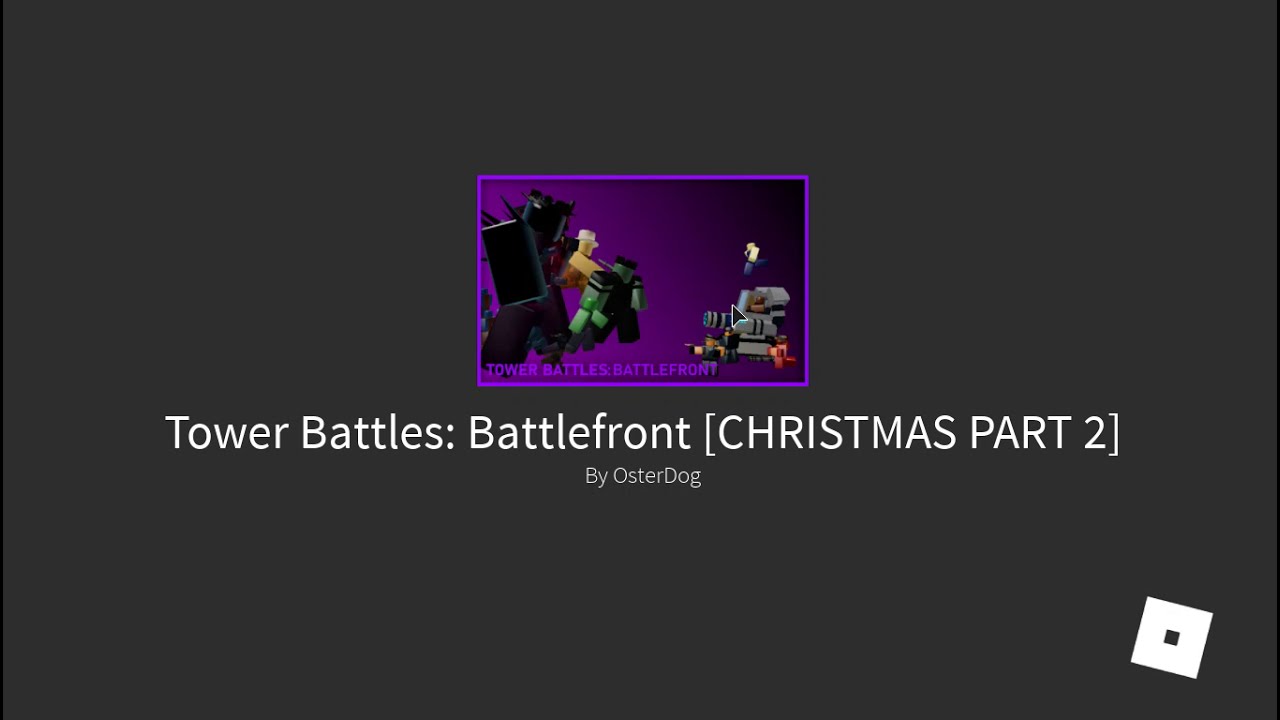The horizontal rectangular image resembles the face of a cell phone with a game interface. The entire background is black. Dominating the center of the frame, bold white text reads "Tower Battles: Battlefront (CHRISTMAS PART 2)." Just beneath this title, in smaller white lettering, it says "By Ostradog.” Above the text is a purple rectangle, which appears to contain a preview image of the game, although specific details are hard to discern due to the image's small size. Within this purple box are figures suggestive of video game action: a dark, possibly menacing robot with green and yellow arms on the left, a female figure, and another robot on the right. In the lower right corner of the frame is a white square tilted at a 45-degree angle, featuring a smaller black square in its center, resembling a stylized logo.